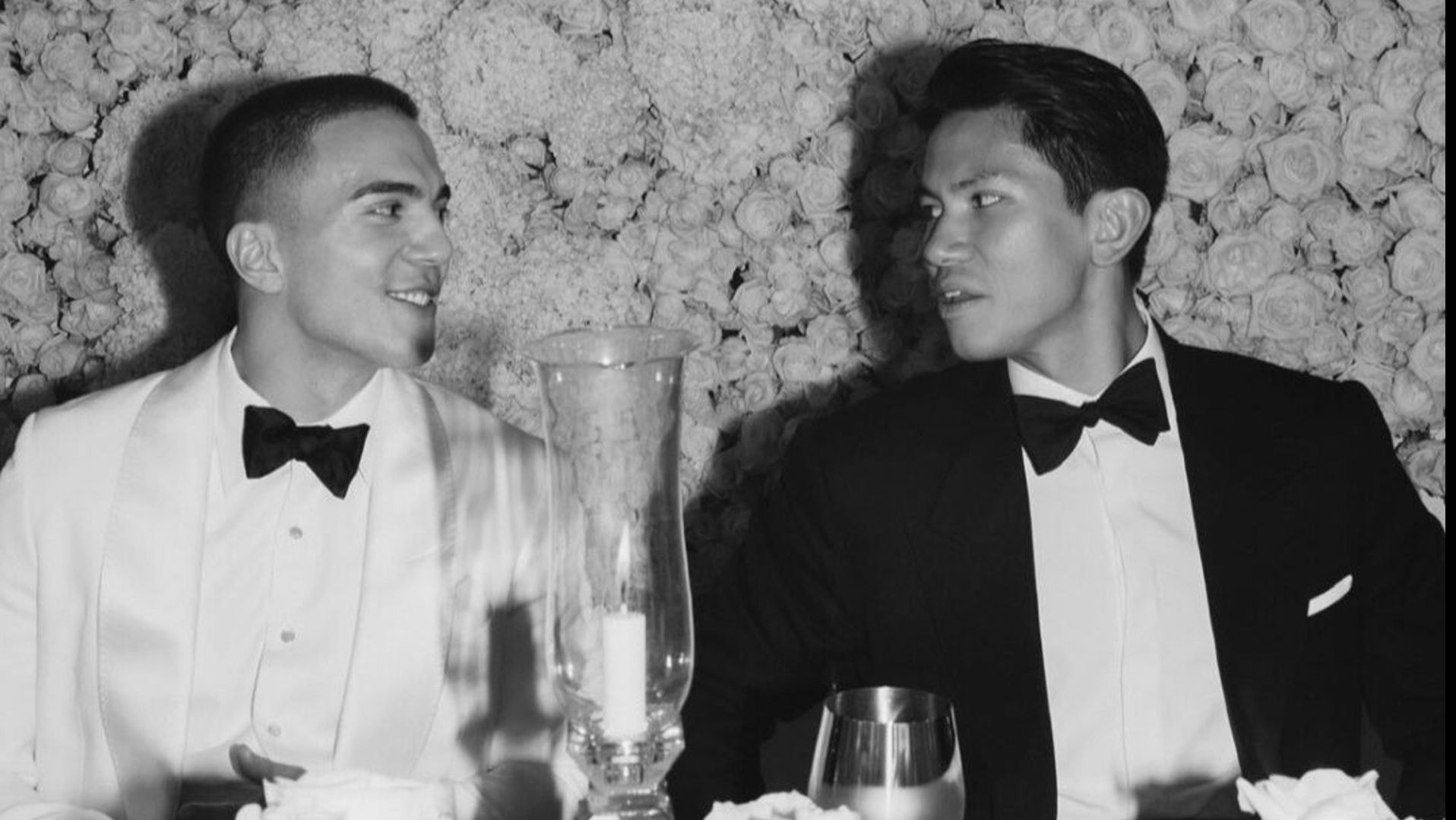This black-and-white photograph, likely from the 1950s, depicts an intimate indoor scene with two young men dressed formally. The man on the right wears a black tuxedo with a white dress shirt and a black bow tie, accentuated by short, thick black hair. The man on the left contrasts him in a white tuxedo, white dress shirt, and also a black bow tie. Between them stands a lit candle encased in glass, casting a warm glow that enhances the elegant ambiance of what appears to be a dinner setting. The table is adorned with a glass containing a clear liquid—possibly water, alcohol, or wine. A small handkerchief peeks out from the breast pocket of the man in the black tuxedo. Behind them, the wall is decorated with a pattern of roses, likely wallpaper, as the photograph being in black and white obscures the true nature of the flowers. Several additional details, like napkins on the table, contribute to the scene's refined atmosphere.